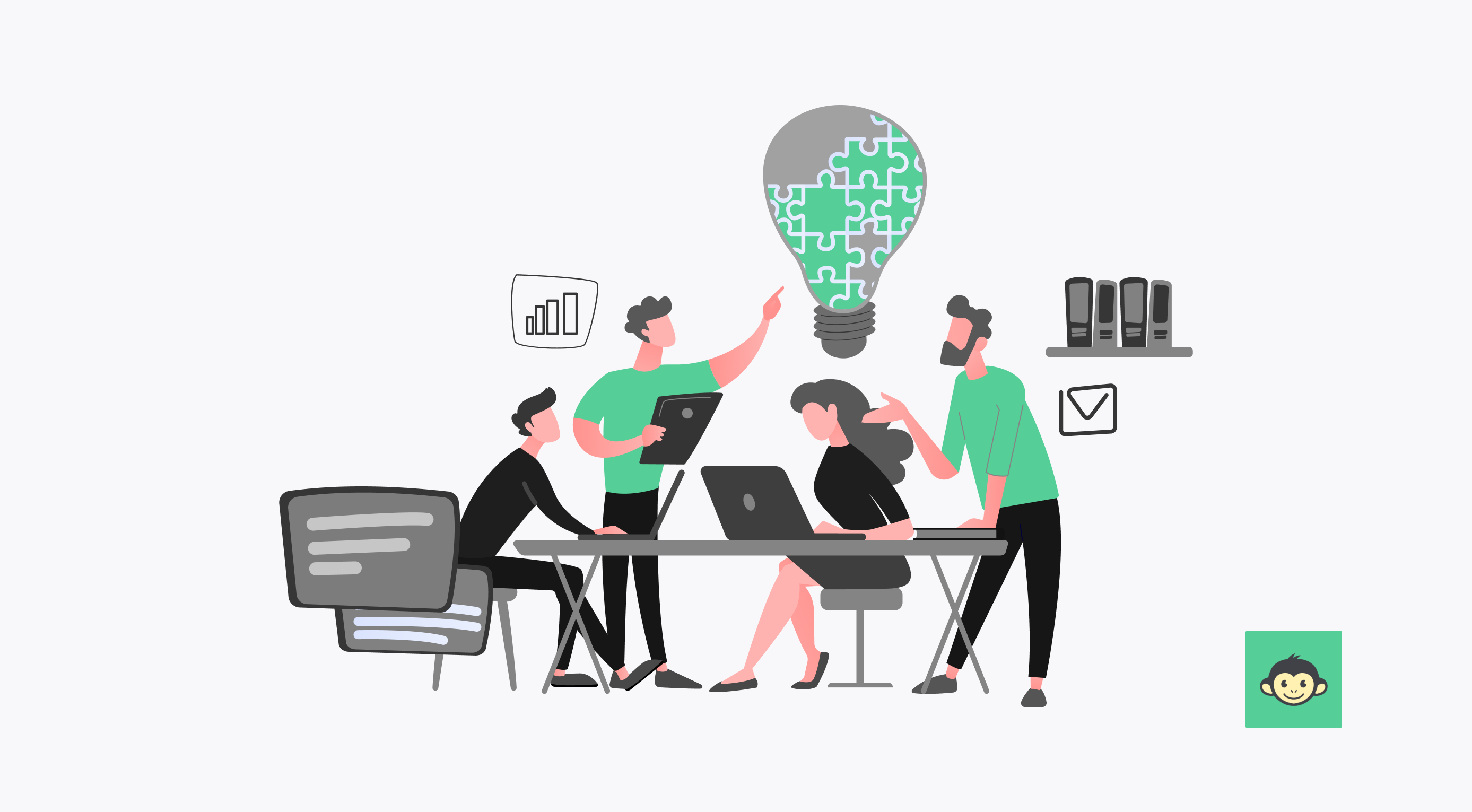A computer-generated, rectangular image showcases a modern workspace with four individuals collaborating at a table. The simplistic, cartoon-like illustration features three men and one woman without facial features. The woman, dressed in a black shirt and skirt, is seated at the table working on a laptop, while a man next to her, also in black attire, works on another computer. 

Two men stand nearby, both wearing green shirts and black pants. One man, noted for his beard and mustache, extends his hand as if making a point. The second man, holding a tablet, points towards a gray light bulb on the wall which has green, partially-filled puzzle pieces. 

The setting is complemented by modern furniture, including a gray seat and a stool. The background is stark white, containing minimalistic details: a gray shelf with four books or possible digital devices, a line drawing of an envelope beneath it, and a small green square in the bottom right corner featuring a monkey’s face, hinting at a possible brand logo. Additionally, one standing man is positioned near a bar graph chart. The overall color scheme emphasizes gray, black, and green.